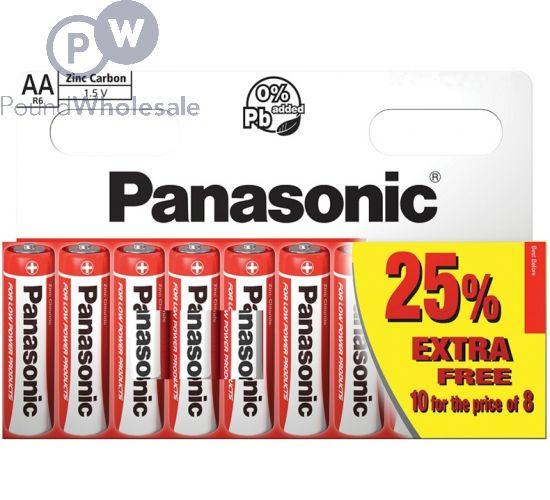This appears to be an advertisement for Panasonic AA Zinc Carbon batteries, highlighted with vibrant and attention-grabbing design elements. 

In the upper left-hand corner, there is an icon that mimics the periodic table, indicating the battery's type as "AA" and its composition as "Zinc Carbon." 

Next to this icon, a circular stamp features the letters "P" and "W," representing "Pound Wholesale," signifying bulk purchase options.

Prominently, in the center, there is another circular icon with a leaf inside, accompanied by the text "0% added Pb," indicating that the batteries are free of added lead.

The central focus of the advertisement is the bold and large "Panasonic®" brand name, showcasing the quality and reliability of the product with the registered trademark symbol.

Beneath this, there is an image of the actual product packaging displaying eight Panasonic batteries.

A striking promotional banner across the top, set against a yellow background, announces "25% Extra Free," and clarifies the offer: "10 for the price of 8."

The advertisement uses a vibrant color scheme primarily consisting of red, yellow, black, white, and gray, making it visually appealing and easy to read.

This detailed visual and text combination leaves a strong impression of the product's value and environmental consciousness.